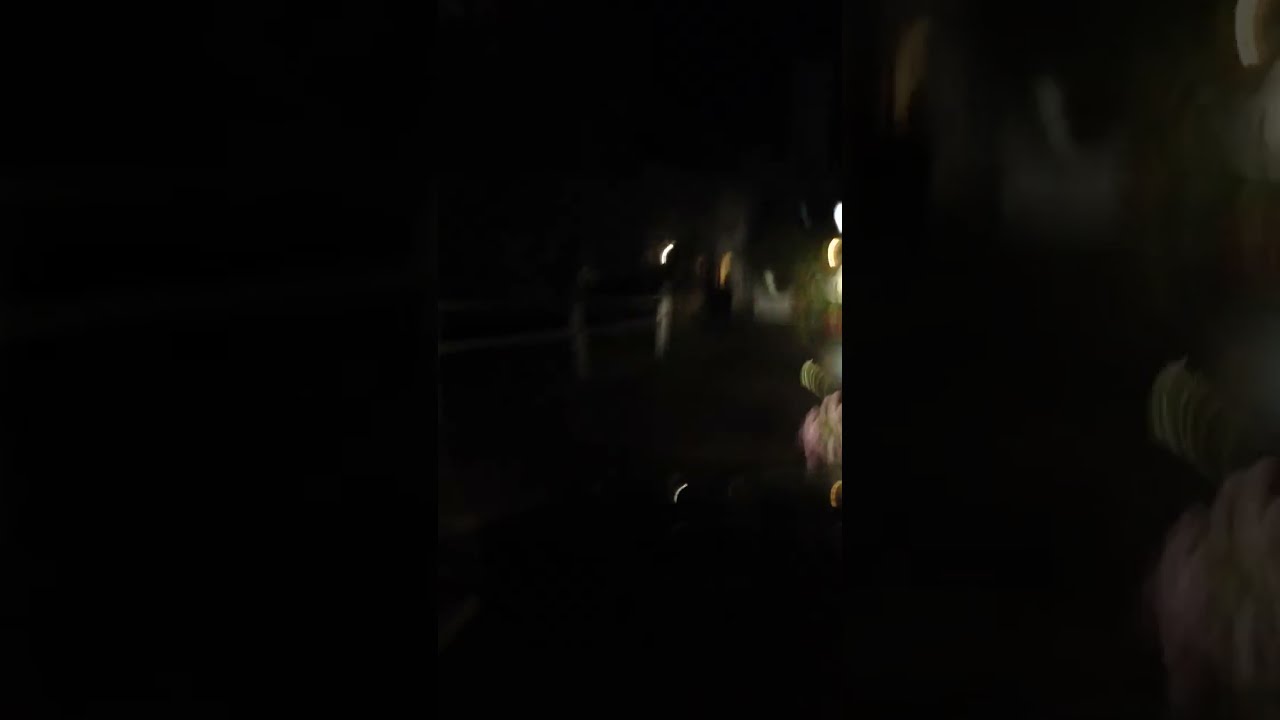This image is a very dark and blurry color photograph in portrait orientation, inset into a darkened landscape-oriented enlargement of the same photograph. The predominant backdrop is mostly black with various indistinct shapes and hints of light. On the right side, you can observe small oval and circular light objects, primarily in greenish, yellowish, and pinkish hues. These brighter shapes are more concentrated towards the top right. A square, too blurred to reveal any details, is situated slightly to the center-right. Scattered light patterns extend toward the left center, further contributing to the sense of motion blur and abstraction. The overall aesthetic resembles photographic representationalism, evoking a modern art effect.